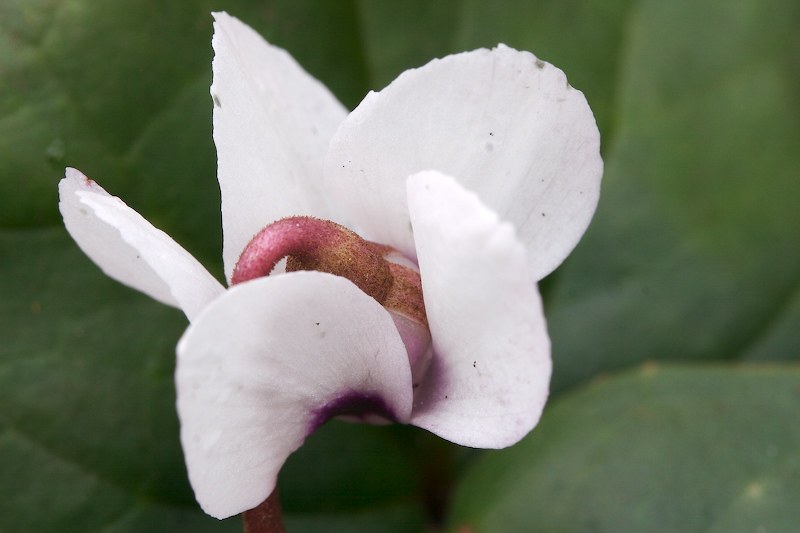The close-up photograph showcases a blooming white flower set against an out-of-focus green leafy background. The flower features five curved white petals, each adorned with patches of purple towards their centers. These petals appear to be in the process of opening, revealing intricate detailing within the flower's core. The center exhibits a striking mixture of colors, including light pink, peach, and brown, with a prominent and distinct purplish-red stamen curving downwards from the middle. This stamen has a slightly hairy texture and exhibits a gradient of brown at its base. Dew droplets can be observed on the out-of-focus leaves in the background, adding to the delicate beauty of the scene. The primary colors in this vividly detailed image include green, white, shades of purple, light pink, and peach.